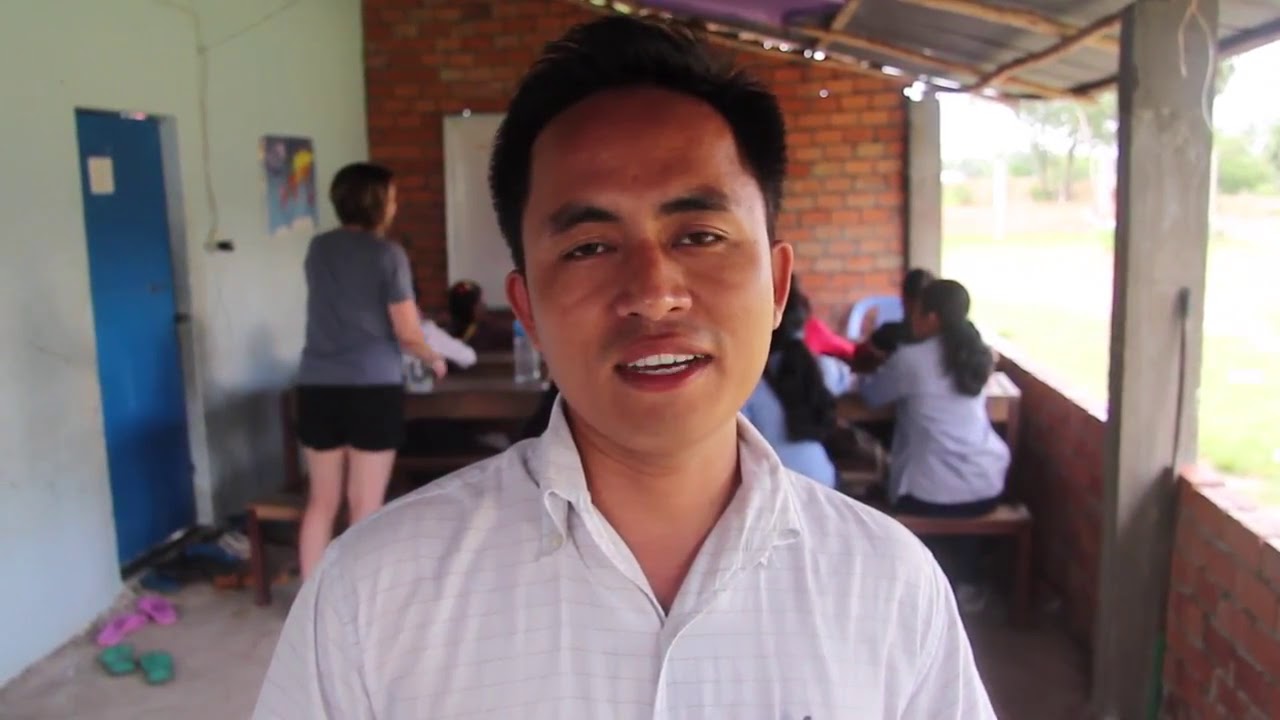In the foreground, a Southern Asian man with dark black hair combed above his forehead stands, looking straight into the camera with slightly squinted brown eyes and a partially open mouth revealing his teeth, as if caught mid-sentence. He wears a white, button-up shirt with horizontal stripes across the collar. To his left, a woman with short brown hair, clad in a gray shirt and black shorts, stands next to a table. Behind the man, to his right, is another group of people seated around a picnic table. Most notably, a woman wearing a long-sleeved white shirt with her black hair pulled back into a ponytail. They are situated under a semi-outdoor structure composed of a brown wooden roof supported by a brown support beam in the middle. The back wall is made of brick, with a closed blue door to the left and an opening to the right that provides a view of grass and trees outside. A waist-high brick wall with a wooden beam on the right separates the indoor area from the outdoors. Additionally, a big wire hangs down the off-white wall on the left, near the blue door. There are scattered items, including people's shoes, inside the door and a bottle of water on the table behind the man's head.